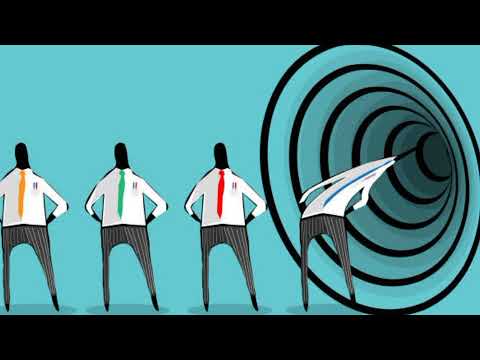The image is a modern, pop art-style color illustration set against a light blue background with black strips across the top and bottom. It features four men positioned in a row, all facing the viewer. Each man is dressed in a white long-sleeve shirt, black pinstripe pants, and a colored tie—gold, green, red, and blue. Their faces are depicted as solid black and they stand with their hands on their hips. On the right side of the image, there is a circular, vortex-like tunnel composed of smaller and smaller circles. The man wearing the blue tie is in the process of being sucked into this tunnel, with his head already entering the funnel's center. The scene is devoid of any text, emphasizing the visual narrative of the figures and the vortex.